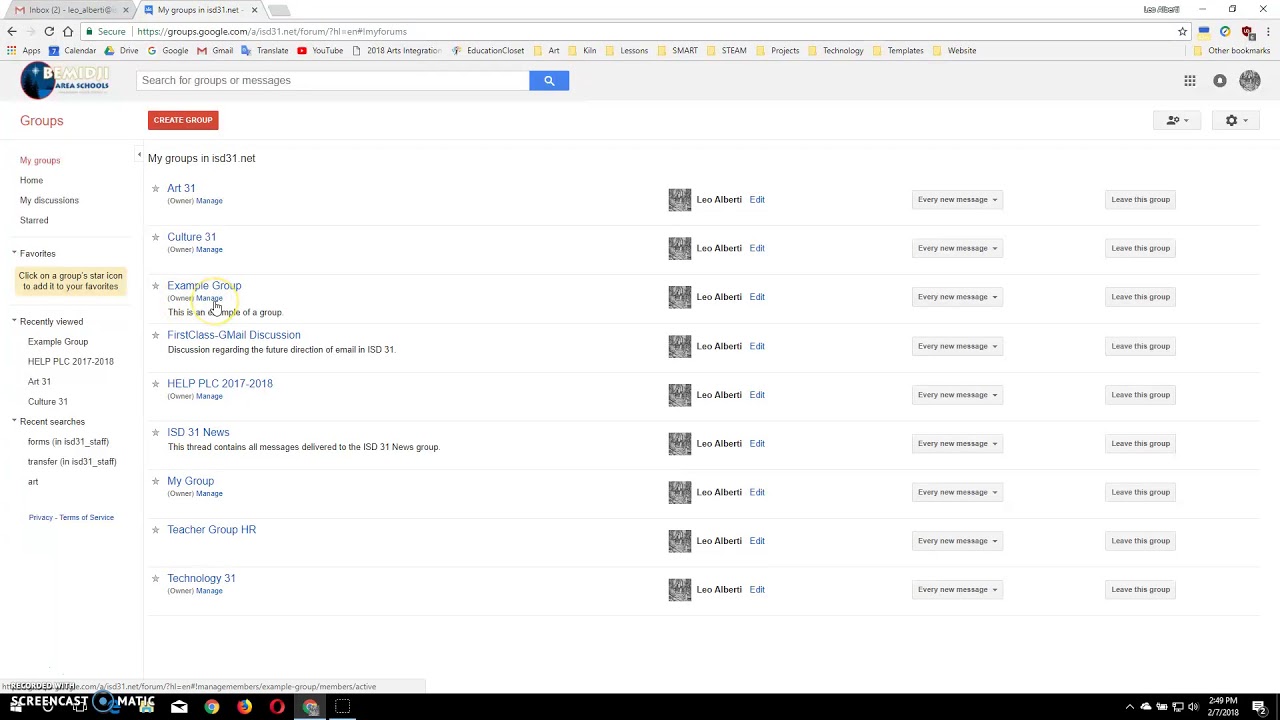In this image, we are viewing a comprehensive screenshot of a web page filled with multiple elements and two open browser tabs. The active tab is from groups.google.com, while the inactive tab is a Gmail inbox for a user named Leo Alberti. 

The browser's interface has a blue logo with "My Groups in ISD31.net" visible, and the standard Windows search bar is present with some pinned apps. The active web page showcases various Google Apps icons in yellow, green, and red, including Gmail, Google Drive, Google Translate, and YouTube.

The web page itself appears to be a Google Groups interface. On the left-hand side, there is a vertical menu that includes options like Groups, My Groups, Home, My Discussions, Starred, and Favorites, along with a message prompting users to click a group’s star icon to add it to their favorites list. Below, there are section headers for Recently Viewed and Recent Searches. Some of the groups listed under Recently Viewed include "Example Group," "Help PLC 2017-2018," "Art 31," and "Culture 31," among others.

A yellow circle with a hand is highlighted over the clickable link for "Example Group" in the center of the page. Each group listed has associated options for "Every new message" and "Leave this group," both of which are clickable. The sidebar also includes folders labeled Art, Film, Lessons, Smart, STEAM, Projects, Technology, and Templates.

At the bottom left of the sidebar is a circular logo that reads "Bemidji Area Schools," featuring a black mountain with a white star and a blue background. The standard Windows taskbar is visible at the bottom of the screen, completing the typical desktop interface.

In summary, the image is a detailed view of a web page displaying Google Groups, featuring various navigation elements, group listings, and user interface components.